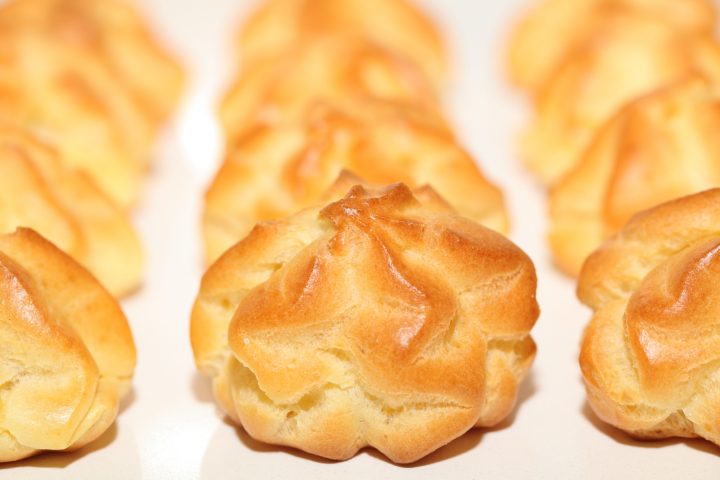The image features a close-up of rows of perfectly baked, bite-sized puff pastries laid out on a white surface, possibly a tabletop or parchment paper. The pastries are arranged in vertical rows that extend from the bottom to the back of the photo, with each row consisting of four to five pastries. The focus is on the center pastry, where you can see its full form, while the adjacent pastries on the left and right are partially visible. Further back, the pastries blur out of focus, emphasizing the depth of field in the image. Each pastry is white and puffy, with a nicely baked, golden-brown exterior showing cracks where the dough has risen. The pastries seem to be uniformly and professionally made, possibly for a bakery. They appear to have been piped with a star tip, giving them an interesting texture. The strong lighting highlights the fine baking details, casting shadows underneath them and accentuating their crispy, flaky layers and toasty finish.